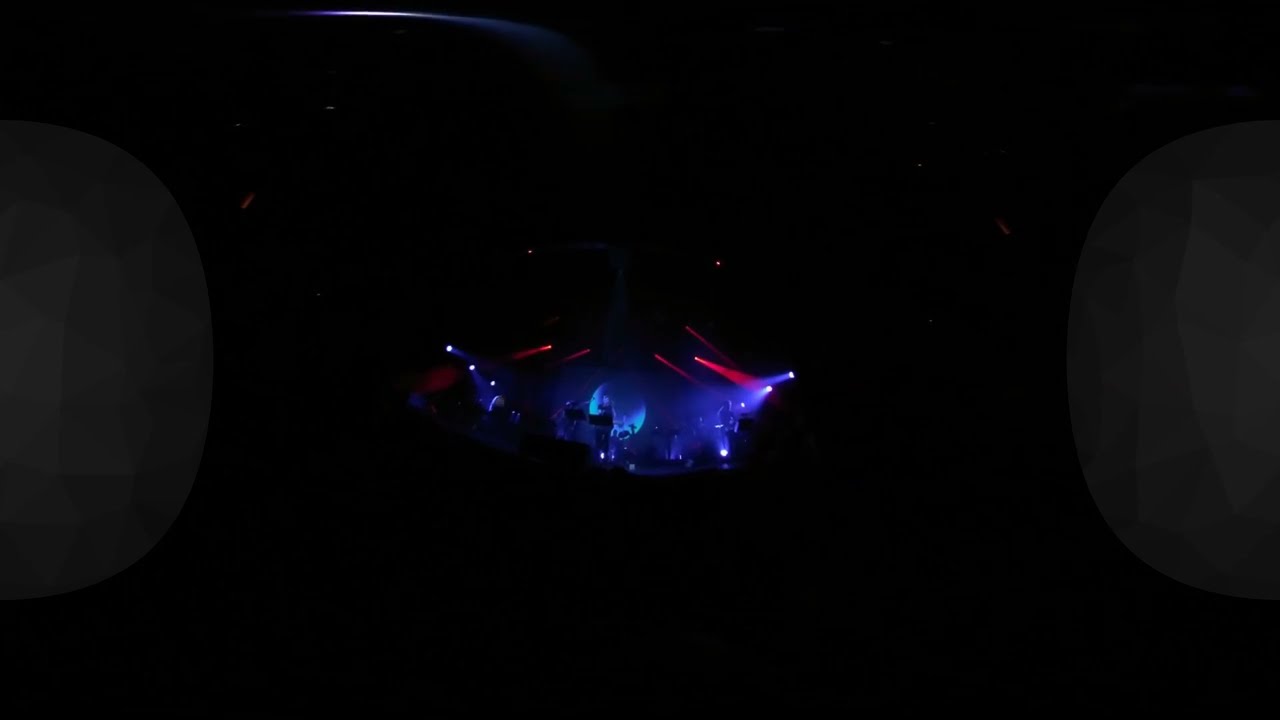The image captures a dimly lit rock concert scene, primarily focused on a stage that dominates the center 10-15% of the frame. The stage is bathed in blue and red spotlights, creating a vivid light show against a backdrop of near-total darkness, where the audience would be. On either side of the image, faint white bubbles resembling fingerprints intrude slightly. The middle of the stage features a mix of blue and purple lights, with some pink streaks adding to the dynamic lighting. Several musicians are discernible: a guitar player on the far right, and possibly a keyboard player and drummer further back, all illuminated by purplish-blue light. The musicians appear to be performing in front of what looks like music or keyboard stands. A circular decoration, which resembles a moon or a 3D-designed gray circle with a diamond-like texture, adds to the mystical ambiance. The primary colors in the image are black, blue, and red, with a hint of white, emphasizing the enigmatic and electrifying atmosphere of the concert.